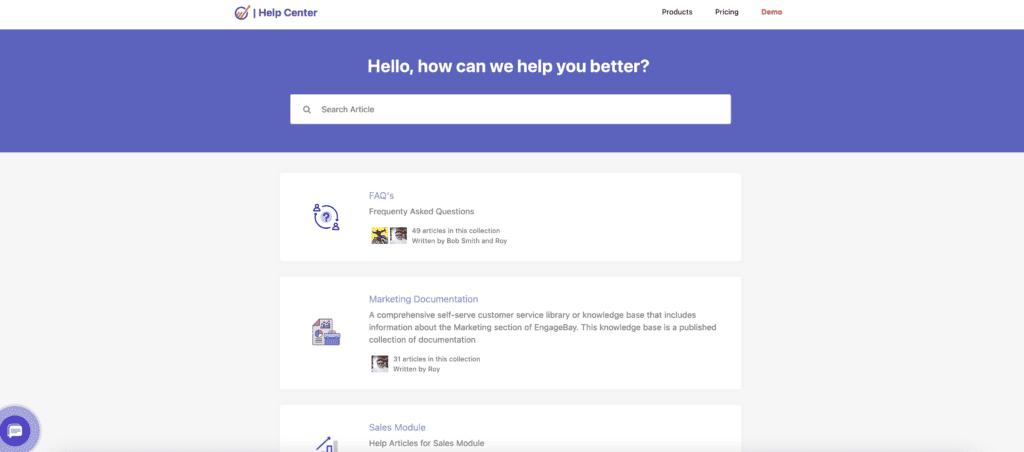The image displays a website help center page with an organized and visually distinct layout.

On the left side, there is a white banner with a purple-colored header labeled "Help Center." On the right side of the banner, there are three options: "Products," "Pricing," and "Demo," with "Demo" highlighted in red.

Below this, a prominent thick purple banner reads "Hello, how can we help you better?" in white font. Directly beneath this banner is a search bar with the placeholder text "Search articles."

The background beneath the search bar is a very light gray, almost white, with several horizontally extended white rectangles serving as content sections.

- The top section is titled "FAQs (Frequently Asked Questions)," containing 49 articles written by Bob Smith and Roy.
- The second section is labeled "Marketing," featuring a comprehensive self-serve customer service library or knowledge base specifically about marketing. This collection includes 31 articles, also authored by Roy.
- The third section, titled "Sales Module," offers help articles related to the sales module; however, the content of this section is partially cut off and not fully visible.

The design employs a clean and structured approach, making it easy for users to find the information they need.